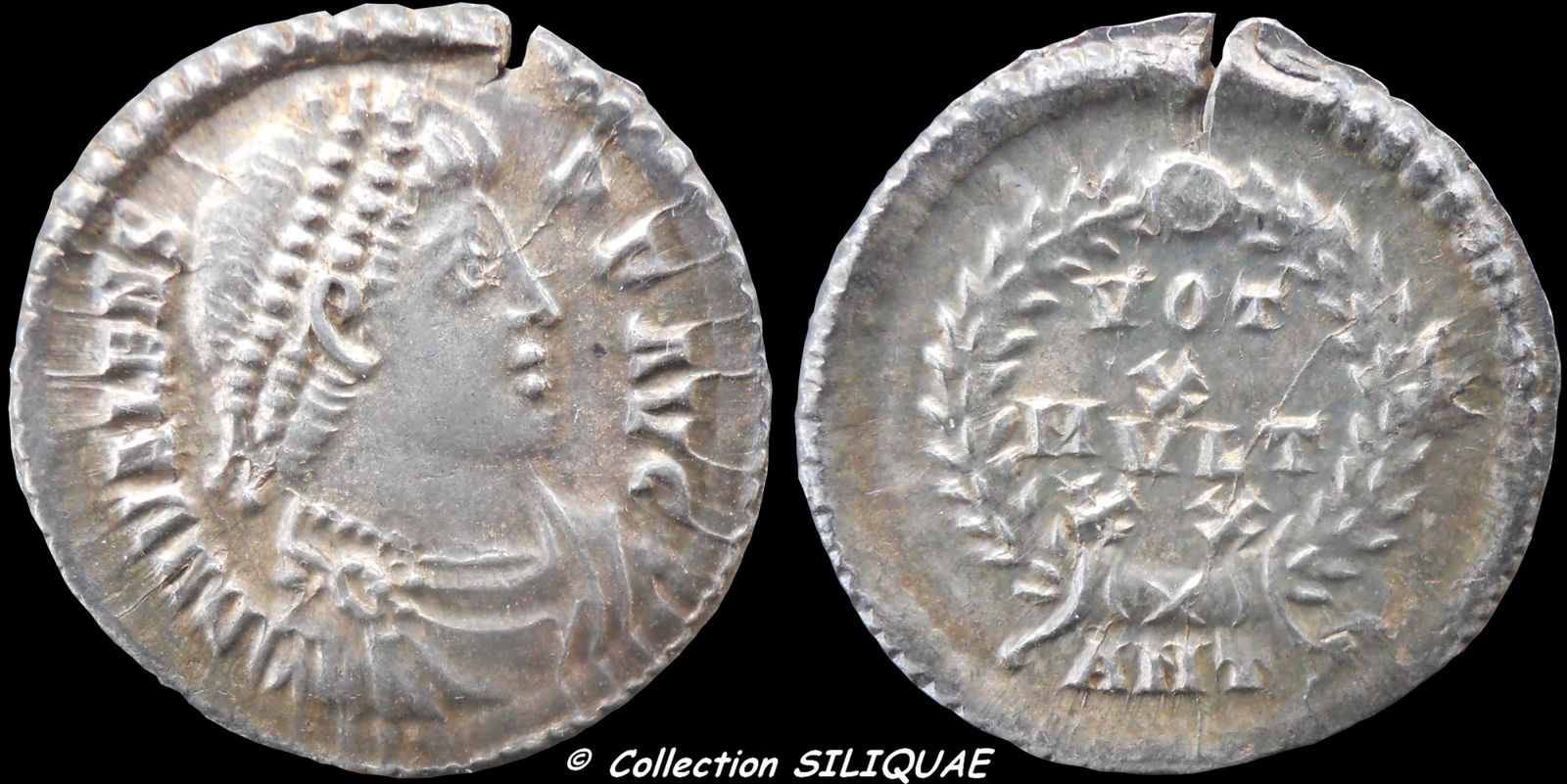This image features a pair of ancient coins, possibly depicting the front and back of a single coin, set against a solid black rectangular background. The left coin displays a right-facing profile of a head, likely a man's, adorned with braided hair or a braided hat. This coin is primarily grayish-brown and shows significant age, with grooves along its ridged edge and a noticeable slit in the upper right part. Both sides of the coin have inscriptions that are difficult to decipher, potentially in Latin. On the right coin, the inscriptions are encircled by a wreath pattern. At the bottom of the image, the text "Collection Siliquae" is prominently displayed in white letters along with a copyright symbol.